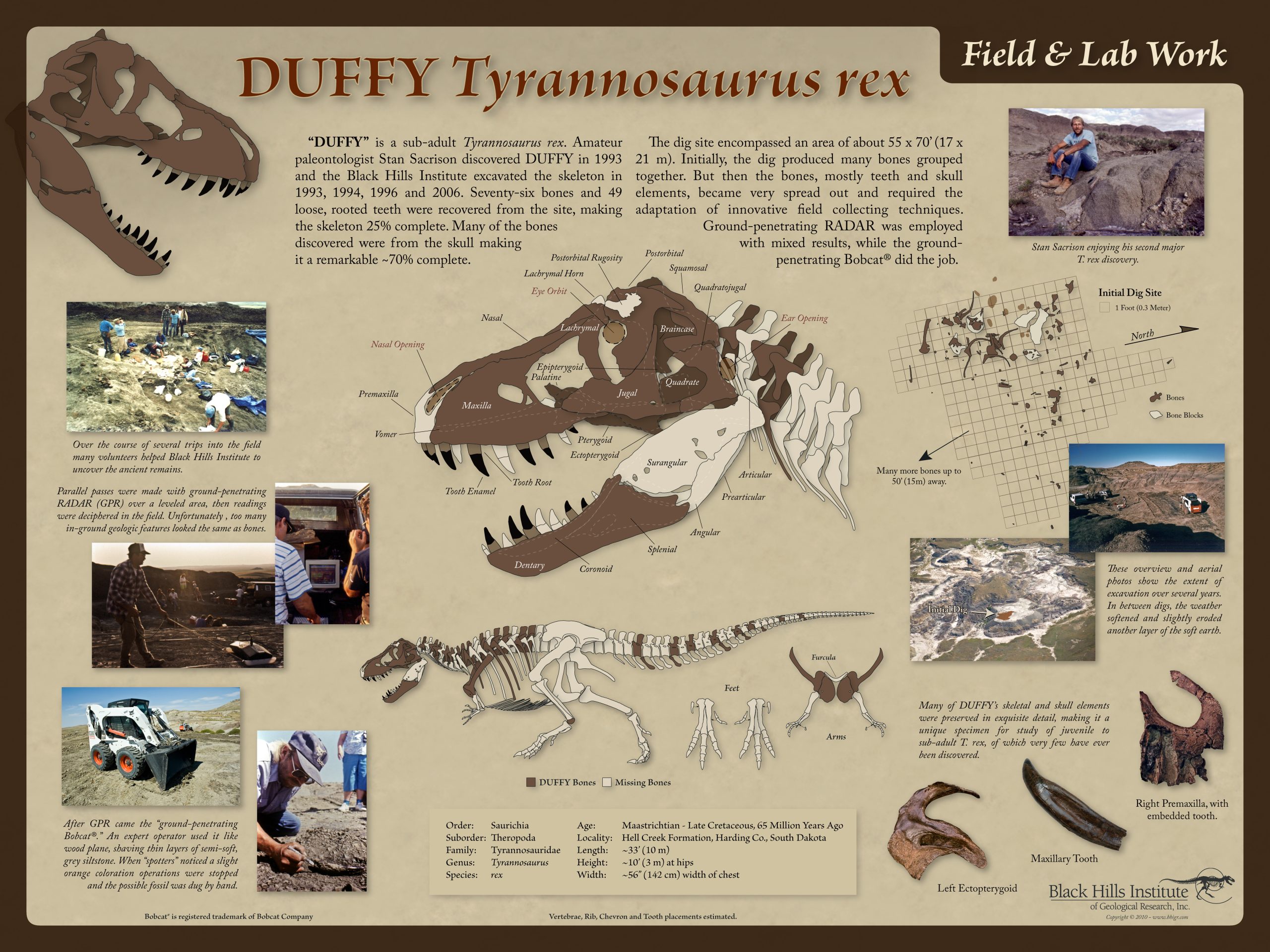This image appears to be from an educational textbook or display panel featuring extensive details about a discovery named "Duffy, the Tyrannosaurus Rex." The overall background is light brown and it is rich with text. At the top, the title reads "Duffy Tyrannosaurus Rex," with "field and lab work" noted in the upper right-hand corner. A computerized illustration of a dinosaur head is prominently featured, detailed with diagrams labeling various parts and structures of the skull.

Accompanying paragraphs discuss the excavation and study of Duffy, an adult Tyrannosaurus Rex discovered in 1993 in the Black Hills. These paragraphs, however, are too small to read clearly. Below the dinosaur illustration, there are pictures of the excavation site, where paleontologists use a large electronic digger to unearth the bones. The photos of the dig site show people at work, though they are too distant to identify clearly. Additionally, there's an individual with short brown hair, wearing blue jeans and a powder blue shirt, sitting barefoot on a rock.

On the left-hand side and the bottom of the image, supplementary photographs further document the excavation process. A site map and associated text give contextual information, including details about the Tyrannosaurus species and mentions of the Black Hills Institute.